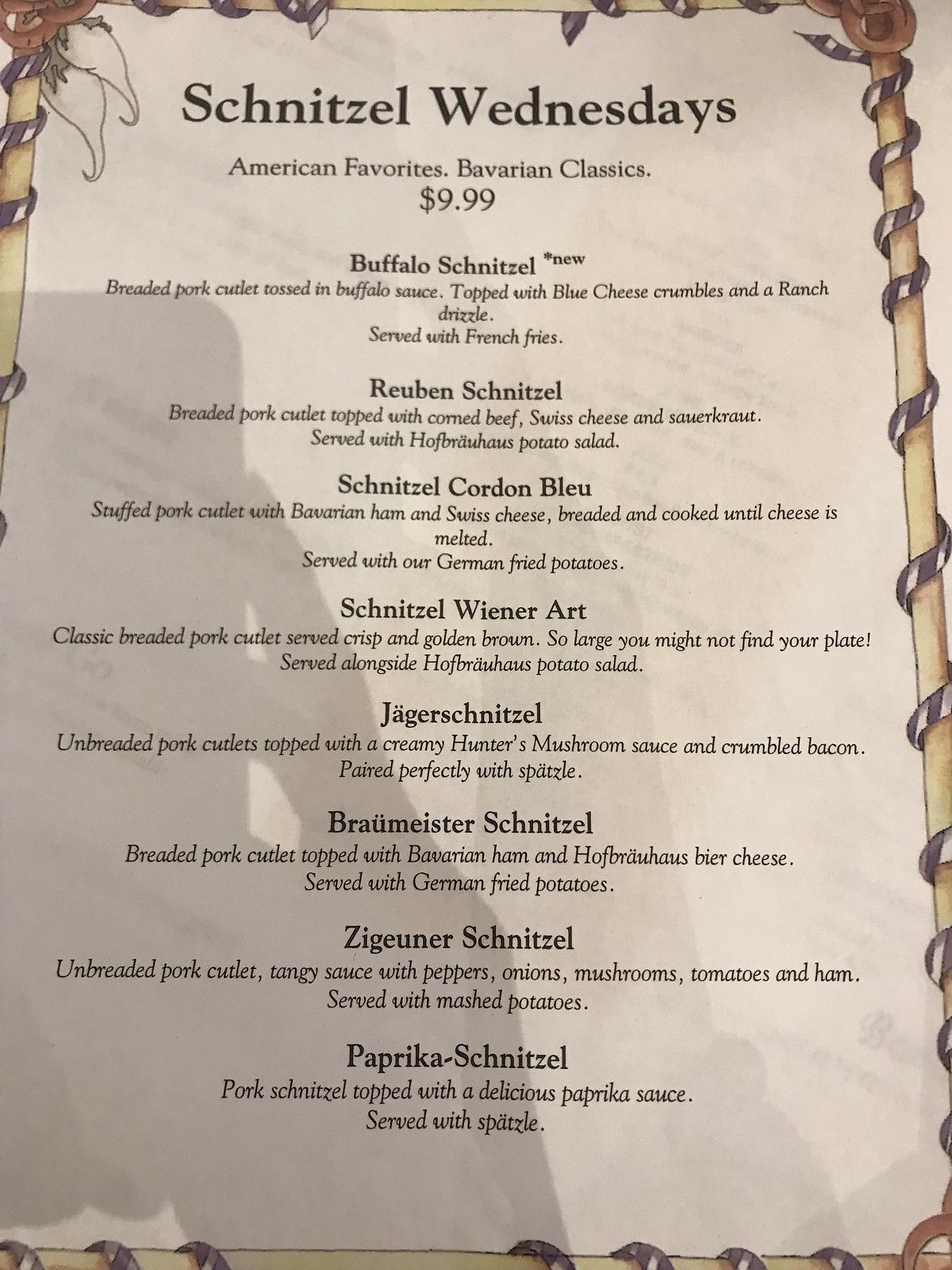The image showcases a restaurant menu titled "Schnitzel Wednesdays." The menu appears to promote a special Wednesday offering that features a selection of schnitzels priced at $9.99 each. At the top of the menu, partial headings can be discerned, reading "American Favorites" and "Bavarian Classics," although some text is blurry. The menu includes various schnitzel options such as Buffalo Schnitzel, Reuben Schnitzel, Schnitzel Cordon Bleu, Schnitzel Wiener Art, Jaeger Schnitzel, Breimeister Schnitzel, Zigeuner Schnitzel, and Paprika Schnitzel. The menu is printed on a white piece of paper with black text, bordered by a brown stick-like frame that has a spiraling vine-like design. Although the restaurant's name is not visible, the extensive selection of schnitzel suggests a German culinary theme. The image focuses solely on the menu, with no additional elements present in the frame.